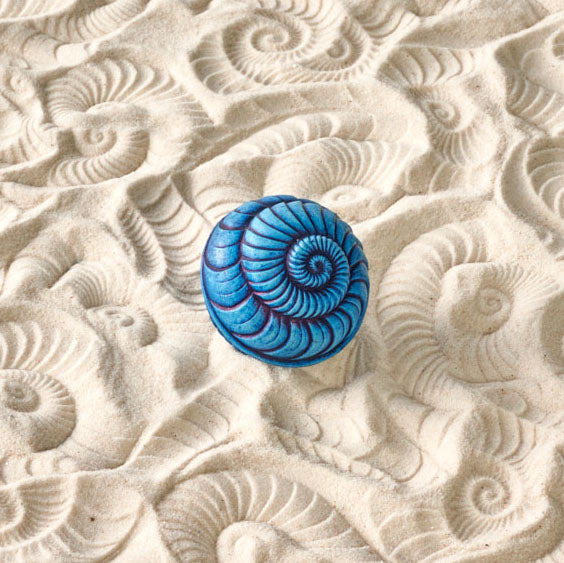In the center of this square image is a beautifully ornamental, fossil-like seashell, characterized by its circular and spiral design with plated layers. The shell boasts a stunning gradient from light blue to darker blue within the rivets of its pattern, accented with hints of purple as it curls inward. Surrounding the shell is a decorative expanse of sand, intricately imprinted with the shell's own design. The sand showcases a range of shades from yellow to light and darker browns, creating subtle shadows that enhance the textured details. The overall setting is serene, dominated by the contrasting hues of blue and yellow, and absent of any text. The shell's spiral design and the matching imprints in the sand evoke an almost fairy-tale-like intricacy, reminiscent of something magical or Disney-esque.